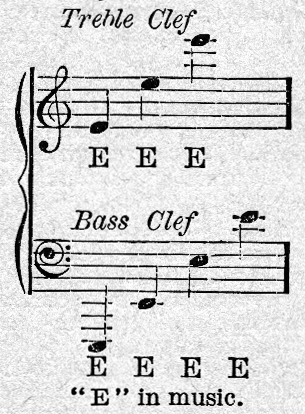The image is a scan of a small section of musical notation set against a grainy background with white and gray speckles. The sheet features two bars, each constructed from five horizontal lines, which serve as the staff. At the top, there is a clear label that says "treble clef," accompanied by the distinctive treble clef symbol. Following this, there are three notes ascending from a lower position to a mid-range and then to a higher note above the staff. Below that, marked "bass clef," another musical sign is present, unfamiliar but suggestive of the bass clef, along with four notes. These notes start very low and ascend gradually, nearing the higher positions seen in the treble clef section. The notes are depicted as teardrop-shaped dots with stems, their orientation and position indicating their pitch within the musical structure.